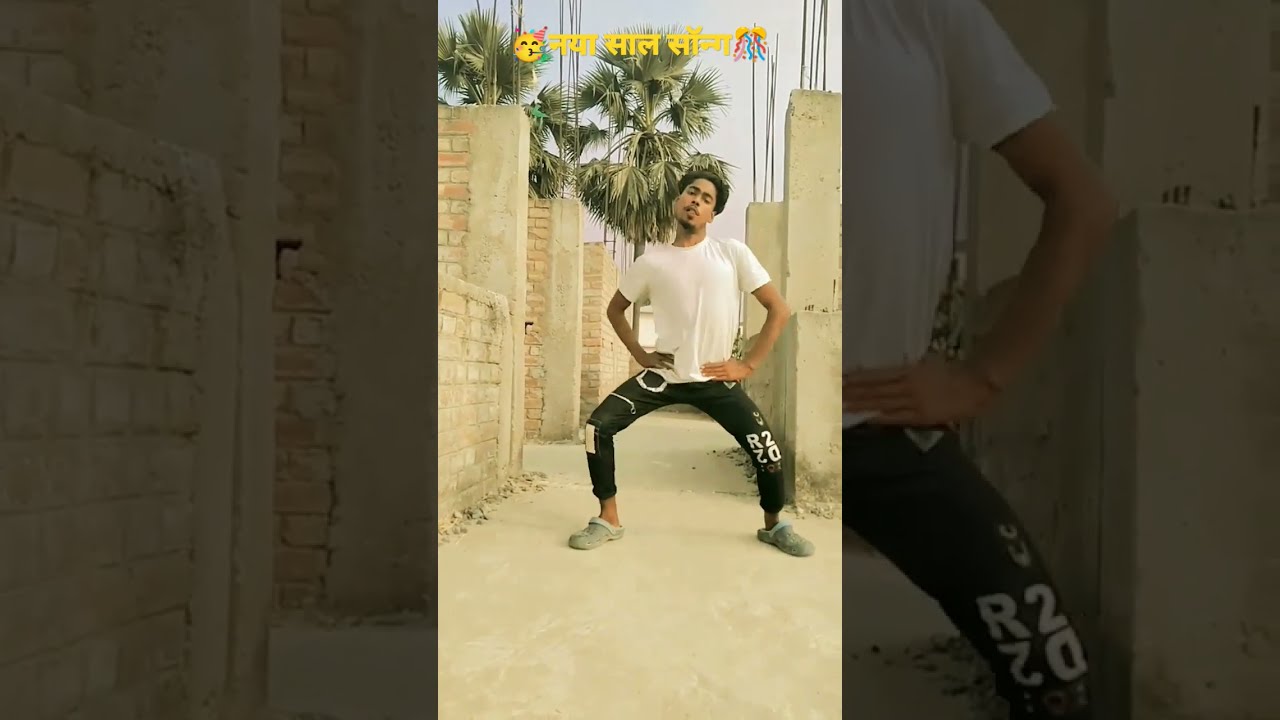The image is divided into three vertical sections. The first and third sections feature a darkened close-up of the central image. The central section displays a detailed outdoor scene. A young man with brown skin, curly black hair, a mustache, a small soul patch, and a faint black beard is captured mid-dance. He is standing in the center of what appears to be a construction site with concrete columns and rebar, alongside a partly visible brick wall. The environment suggests an incomplete building with a ground composed of sand and concrete.

The man is wearing a white short-sleeved t-shirt, black pants, and grey slippers or Crocs. His dancing stance includes his hands placed firmly on his hips, legs spread wide and bent at the knees, and his head tilted to the side. He appears to be puffing out his chest, adding to his animated expression. In the background, several palm trees are visible, and it appears to be an overcast day.

At the top corner of the image, there is text in Hindi that reads "Nayasalsong," flanked by two emojis, one of which seems to be a birthday emoji.